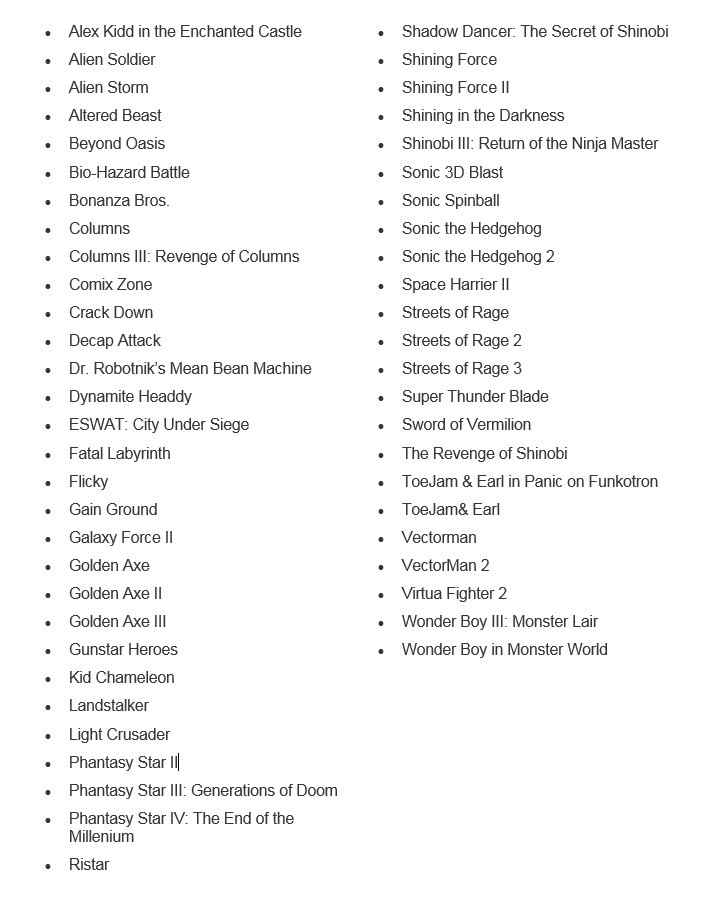A screenshot of a computer screen displays an extensive list of video game titles organized alphabetically. The list begins at the top left corner, with each game prefixed by a bullet point and continues in a single column that extends downward before spanning to the right side of the image. 

At the beginning of the list, the first title reads "The Kid in the Enchanted Castle," followed by an array of other game titles: "Alien Soldier," "Alien Storm," "Altered Beast," "Beyond Oasis," "Bio-Hazard Battle," "Bonanza Bros," "Columns," "Columns II," "Revenge of Columns," "Comix Zone," "Crack Down," "Decap Attack," and so forth. 

Further down, notable entries include "Dr. Robotnik's Mean Bean Machine," "Dynamite Headdy," "ESWAT: City Under Siege," "Fatal Labyrinth," "Flicky," "Gain Ground," "Galaxy Force II," "Golden Axe," "Golden Axe II," and "Golden Axe III." 

The list seems meticulously ordered in alphabetical sequence, with titles like "Kid Chameleon" appearing in the middle and progresses sequentially until reaching 'W'.